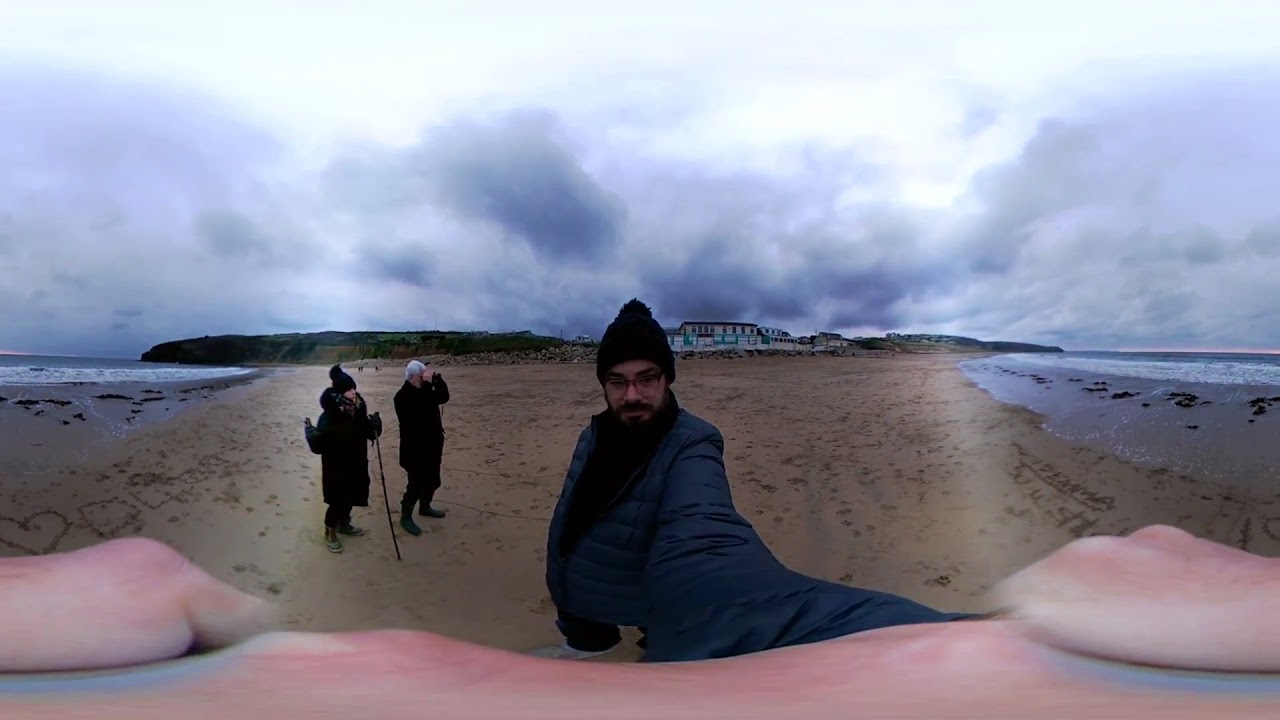In this detailed image, a man is capturing a selfie on a gloomy day at a beach, using a 360-degree camera that produces a warped fisheye effect. He is dressed in a navy blue puffer jacket and a black knit cap, with glasses, and a black mustache and beard. The beach scene showcases sand with a light tan color, flanked by water on both sides, suggesting a narrow strip of land or a peninsula. 

To his left, an elderly man with white hair, wearing a black coat and holding binoculars, peers towards the right. Next to him sits a woman in a black knit coat and pants, holding a walking stick. In the sand beside the woman, there is a heart drawn, possibly inscribed with an unreadable name.

The background reveals a teal, yellow, and brown-roofed building that resembles a house. The sky above is overcast with dark, water-saturated clouds, and sunlight intermittently breaking through. The scene also includes distant shorelines and a rock wall with green foliage, adding to the natural, moody atmosphere of the image.